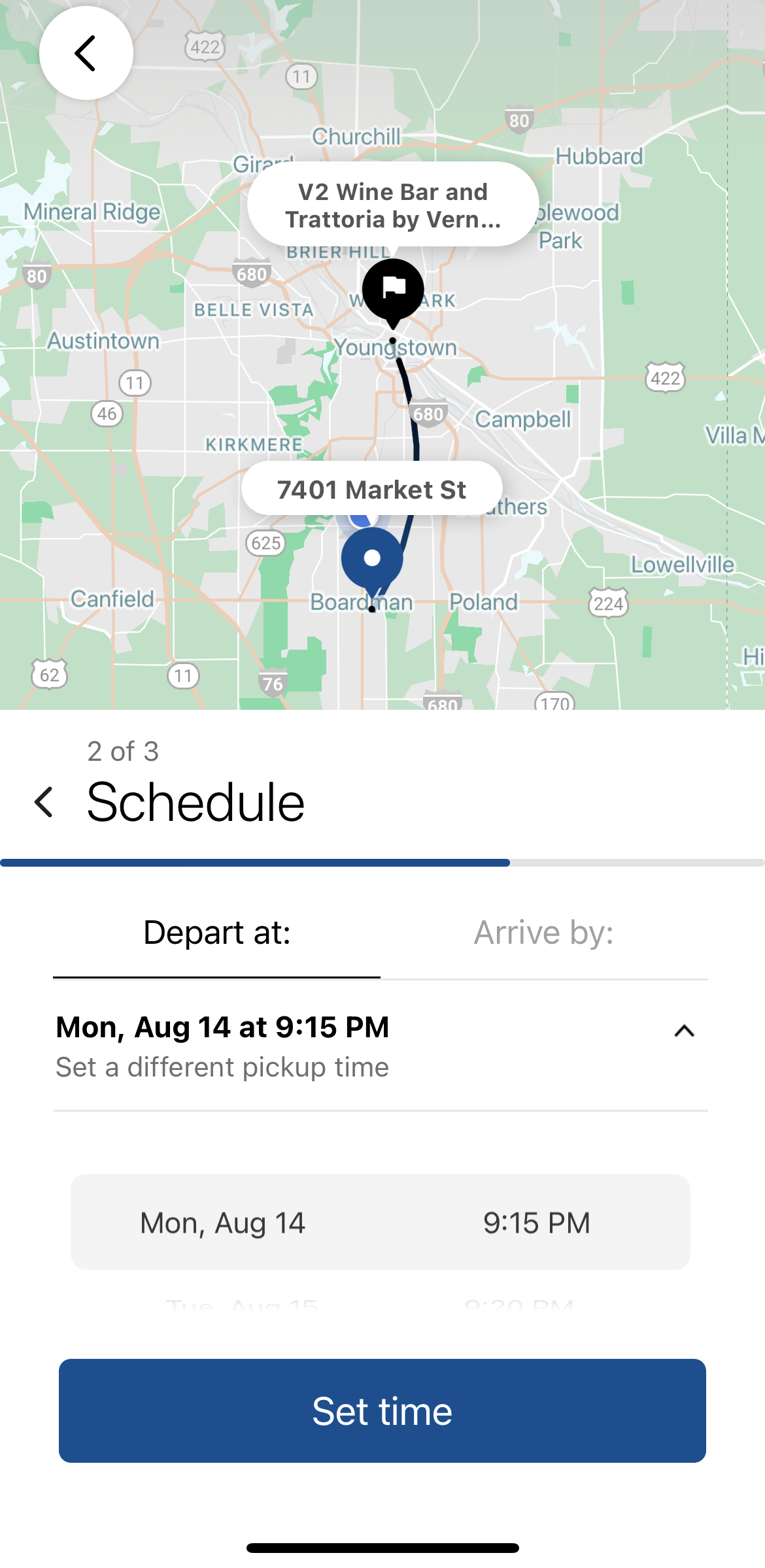In this image, we see a detailed screenshot from a map service interface. The upper half displays a map with notable markers. At the lower section of the map, there's a blue pin-like circle with a white dot in its center, representing a location, identified in an adjacent bubble as "7401 Market Street." A black line runs from this circle to another point at the map's center, which is marked by a black circle with a white flag and labeled "V2 Wine Bar and Trattoria by Verne."

In the top-left corner of the map, there is an arrow inside a white circle, pointing left, presumably for navigation. 

Moving to the lower half of the image, we see the scheduling interface. In the top-left corner, the word "Schedule" is prominently displayed with “2 of 3” above it and a left-pointing arrow. Directly below "Schedule," a detailed progress bar stretches horizontally, with a blue segment filling approximately 60% of its length. 

Further down, the words "Depart at" and "Arrive by" are shown on the left, with their respective times "Monday, August 14th at 9:15 PM" beside them. Next to the time, there is an upward-pointing arrow. At the very bottom of the image, the option to "Set Time" is available.

This description highlights the key map labels, the scheduling information provided, and the various interface elements present in the image.